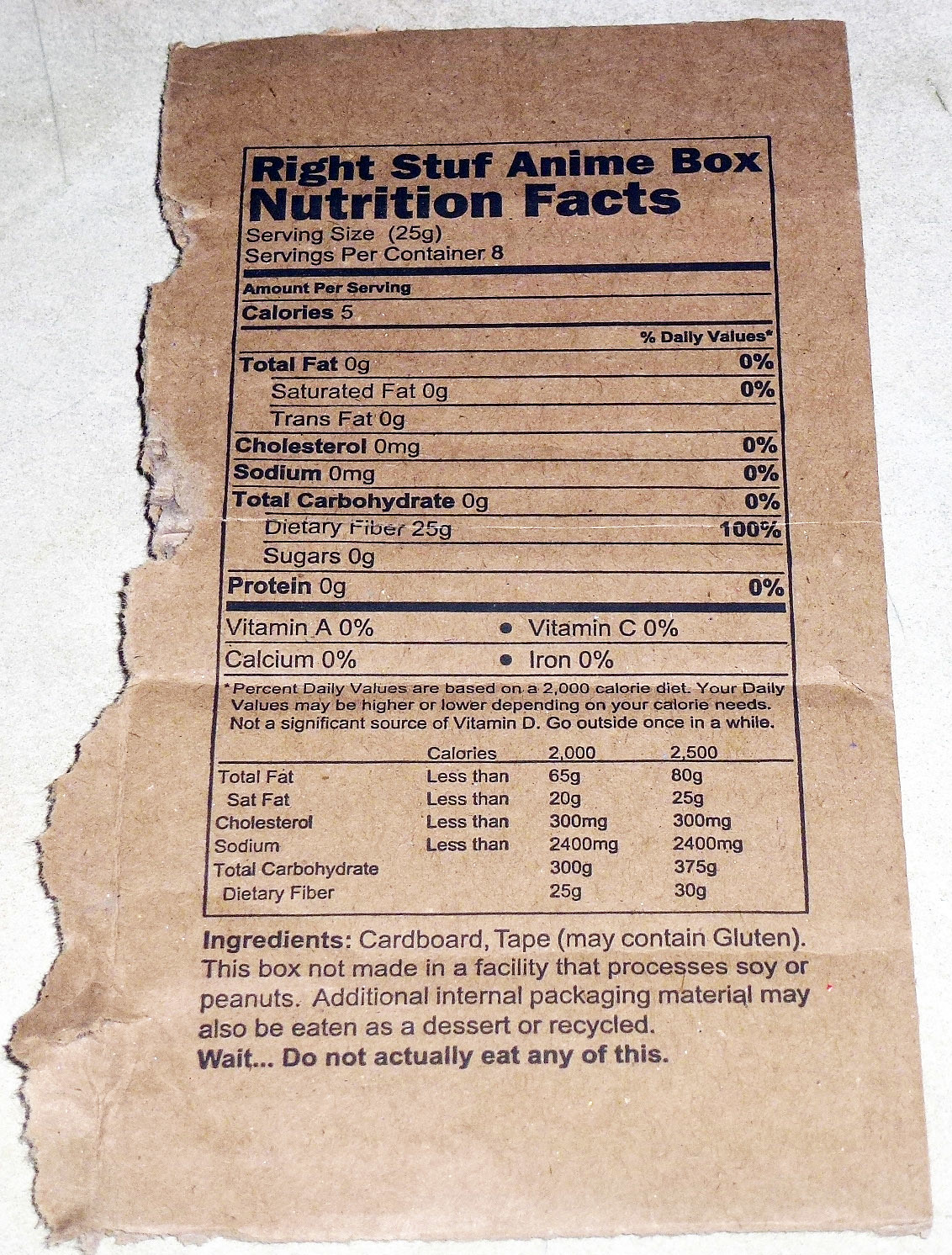This photograph features a torn section of a cardboard box displaying the Nutrition Facts label. The label is set against a flat, grayish-white surface with a slightly rough texture, likely granite. The torn edges of the label on the left are noticeably jagged, indicating it was ripped from the original packaging. The cardboard label itself is brown, with the upper half being darker and the lower half being lighter in shade. In the middle of the label is a large black rectangle containing the Nutrition Facts, printed in dark blue text within a thin blue outline. The text starts with the header "Write Stuff Anime Box Nutrition Facts," with a noticeable typographical error in "Write Stuff" using only one "f." 

Detailed information listed on the label includes:

- Serving Size: 25 grams
- Servings Per Container: 8
- Calories: 5
- Total Fat: 0 grams
- Saturated Fat: 0 grams
- Trans Fat: 0 grams
- Cholesterol: 0 milligrams
- Sodium: 0 milligrams
- Total Carbohydrates: 0 grams
- Dietary Fiber: 25 grams
- Sugars: 0 grams
- Protein: 0 grams

Percent Daily Values for Vitamin A, Calcium, Vitamin C, and Iron are all at 0%. The label appears to be humorous, listing "Cardboard and Tape" as the ingredients, further suggesting that this might be a joke or novelty item.